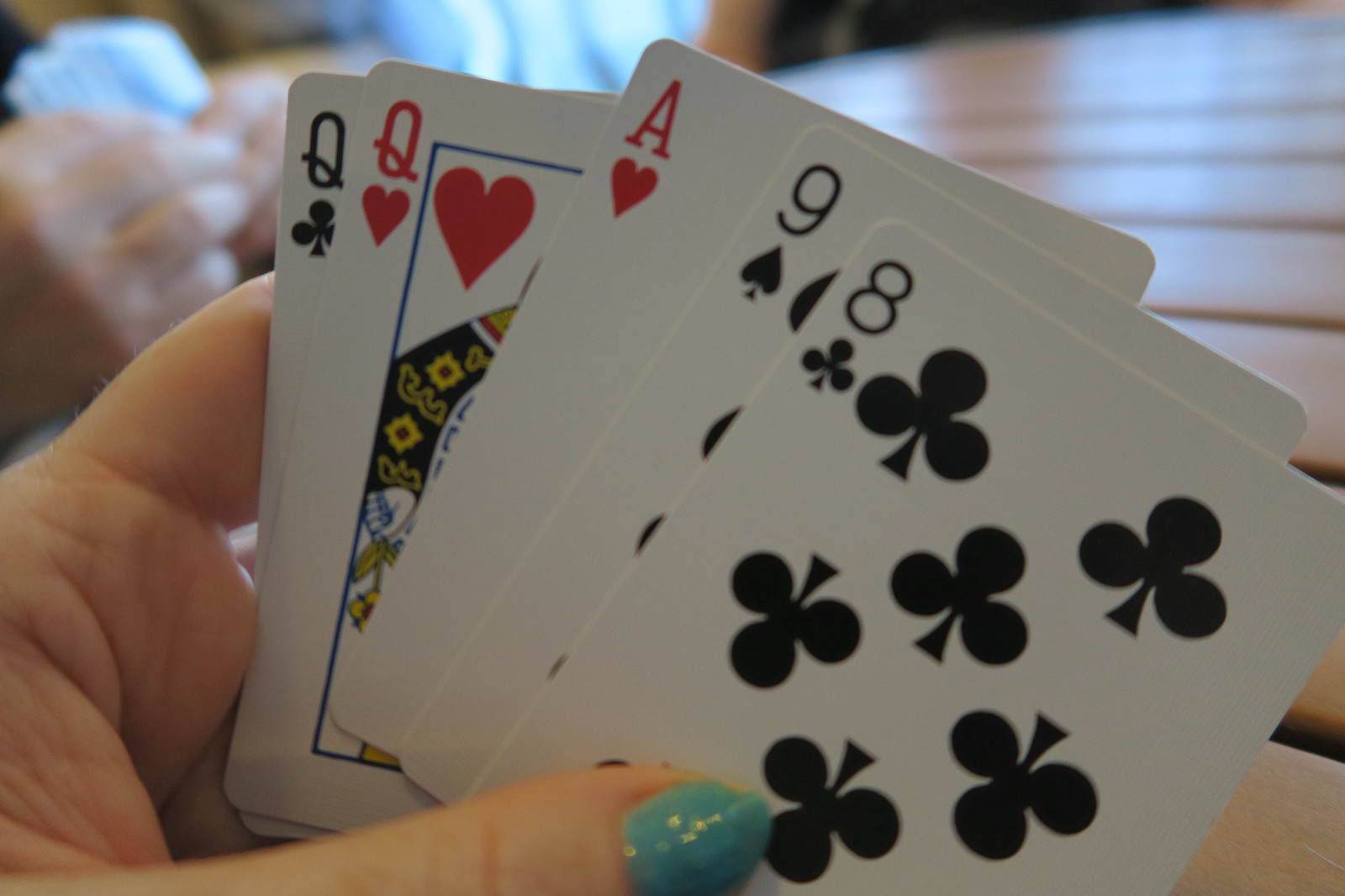In the image, a person’s left hand is prominently featured, holding a five-card hand of traditional playing cards. The visible portions of the hand include the thumb, forefinger, and a bit of the palm, with the other fingers obscured by the cards. The playing cards are displayed in the following order from left to right: Queen of Clubs, Queen of Hearts, Ace of Hearts, Nine of Spades, and Eight of Clubs. Notably, the Queens sit adjacent to each other, while the Ace of Hearts slightly protrudes, making it the most visible card. The Nine of Spades and Eight of Clubs are spaced equidistantly apart, with the Eight being fully visible. 

The setting appears to be a wooden-slatted table where the cards are rested. To the left of the main hand, two additional hands, presumably from another player, also hold their cards, though the card backs are visible and their pattern is indistinct. 

Illumination is sourced from a light coming from the opposite direction of the cardholder, casting reflections off the table's surface. The hand appears slightly wrinkled, suggesting it might belong to an older person. The visible thumbnail is shaped pointedly and painted light blue with sparkly colors, capturing some of the light’s reflection. The remaining fingernails are concealed by the cards. The entire scene exudes a sense of anticipation and strategy inherent to the game being played.